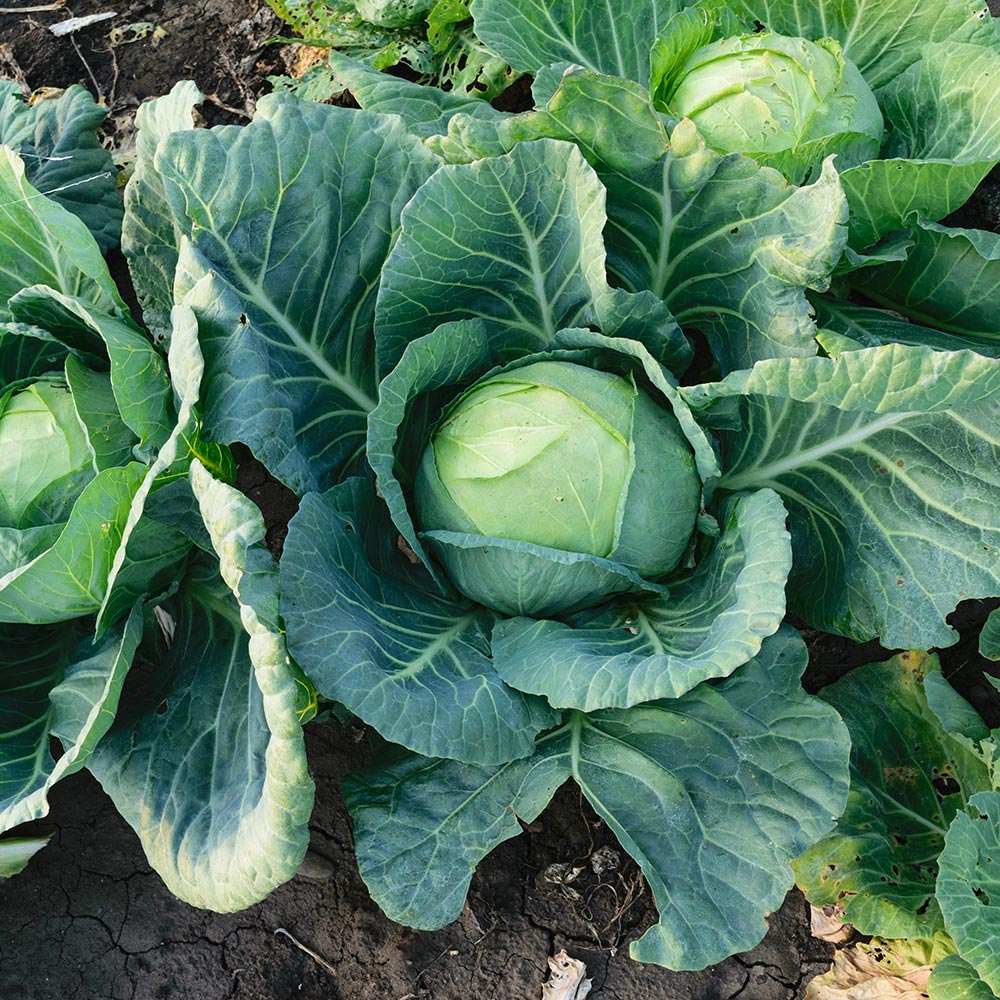This top-down, close-up image depicts a thriving cabbage garden with multiple heads of cabbage surrounded by very large, overlapping green leaves. Dominating the center of the photo is a prominent green and white cabbage head, ready for harvest. Surrounding this central cabbage, several more heads can be seen—one in the upper right corner, another along the lower right, and a smaller one emerging in the left center. The soil, a deep brown to black color, appears at the edges, particularly noticeable in the upper left and bottom left corners, along with scattered patches throughout the image. The cracked, dry texture of the soil suggests recent exposure to the sun, possibly taken during morning or evening. The cabbages are planted very closely, with the giant leaves touching each other and creating a lush, dense foliage that fills the nearly square frame of the photograph.